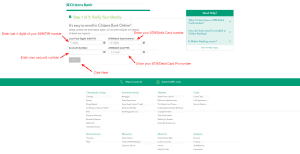This image appears to be a screenshot of a cluttered and densely filled interface, likely from a software application or a document. The image is notably small and illegible. A bold green bar horizontally bisects the image, separating it into a top and bottom section. 

In the bottom section, there are multiple columns of extremely small black text. The text is so tiny that it is unreadable and no specific content can be distinguished.

The top section contains more black text, prominently featuring a green heading. A smaller green sub-bar is positioned to the right within this section. Some of the text on the top part is annotated with red remarks and arrows, seemingly to highlight or specify certain parts of the content. Additionally, there is a grey button located at the bottom of the top section, though its purpose or label is unclear due to its minuteness.

Overall, the image is highly detailed yet impossible to decipher due to its diminished scale, leaving its exact nature and content indeterminable.